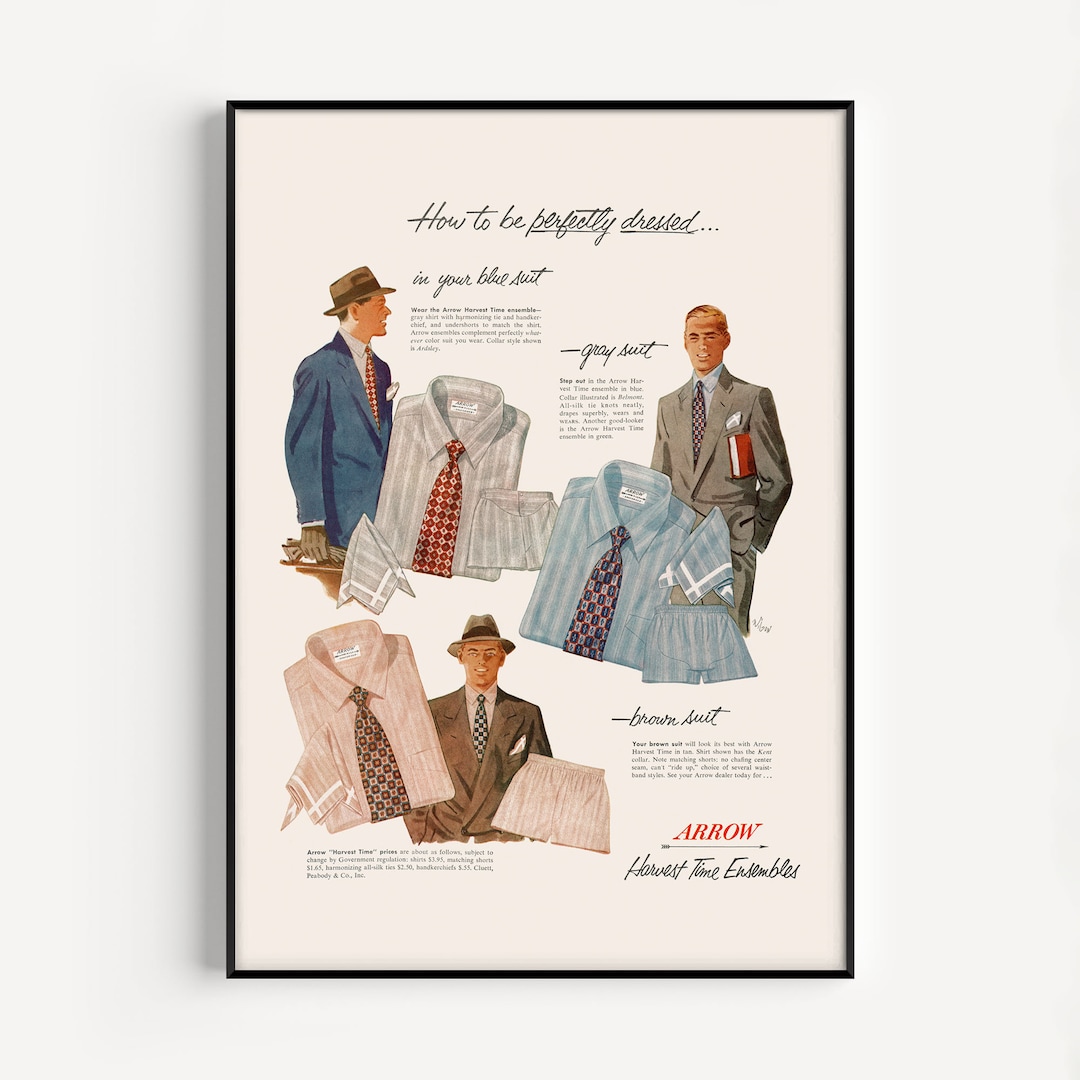The image is a framed advertisement, likely from the 1940s or 1950s, featuring three men dressed in business suits, each showcasing different ensembles from Arrow's "Harvest Time Ensembles" collection. The men appear proper and polished, illustrating how to be perfectly dressed in each suit. The man on the left is wearing a blue suit paired with a gray shirt, boxer shorts, a handkerchief, and a red and gold tie. The man in the middle, dressed in a gray suit, matches it with a blue and light blue striped shirt, boxer shorts, a pocket square, and a blue, red, and gold tie. The man on the bottom, clad in a brown suit and a hat, complements his look with a light pink shirt, boxer shorts, a pocket square, and a tie adorned with gold and red accents. Folded images of the suits in blue, pink, and gray accompany the advertisement, further illustrating the stylish ensembles. At the bottom of the image, the text reads, "Arrow Harvest Time Ensembles."